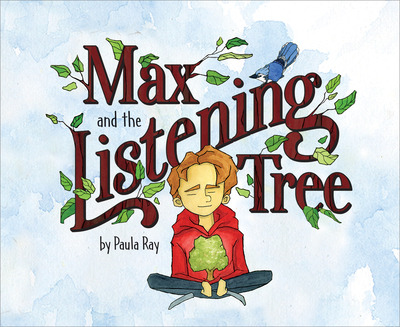The cover of the children's book titled "Max and the Listening Tree" by Paul Bray is an engaging and whimsical illustration featuring an aquarelle-style blue background with various shades of blue. The book's title, "Max and the Listening Tree," is prominently displayed in the center using deep brown lettering that mimics a wooden texture, with small green leaves growing out of the letters. Perched on the final letter of "Listening" is a delicate little bluebird. Below the title is an illustration of a young boy with blondish hair and a fair complexion, sitting cross-legged. He is wearing a bright red hoodie adorned with a tree graphic, complemented by gray pants. The cover combines colors such as blue, brown, green, red, gray, and flesh tones to create a visually appealing and easy-to-read design, characteristic of high-quality children's books.